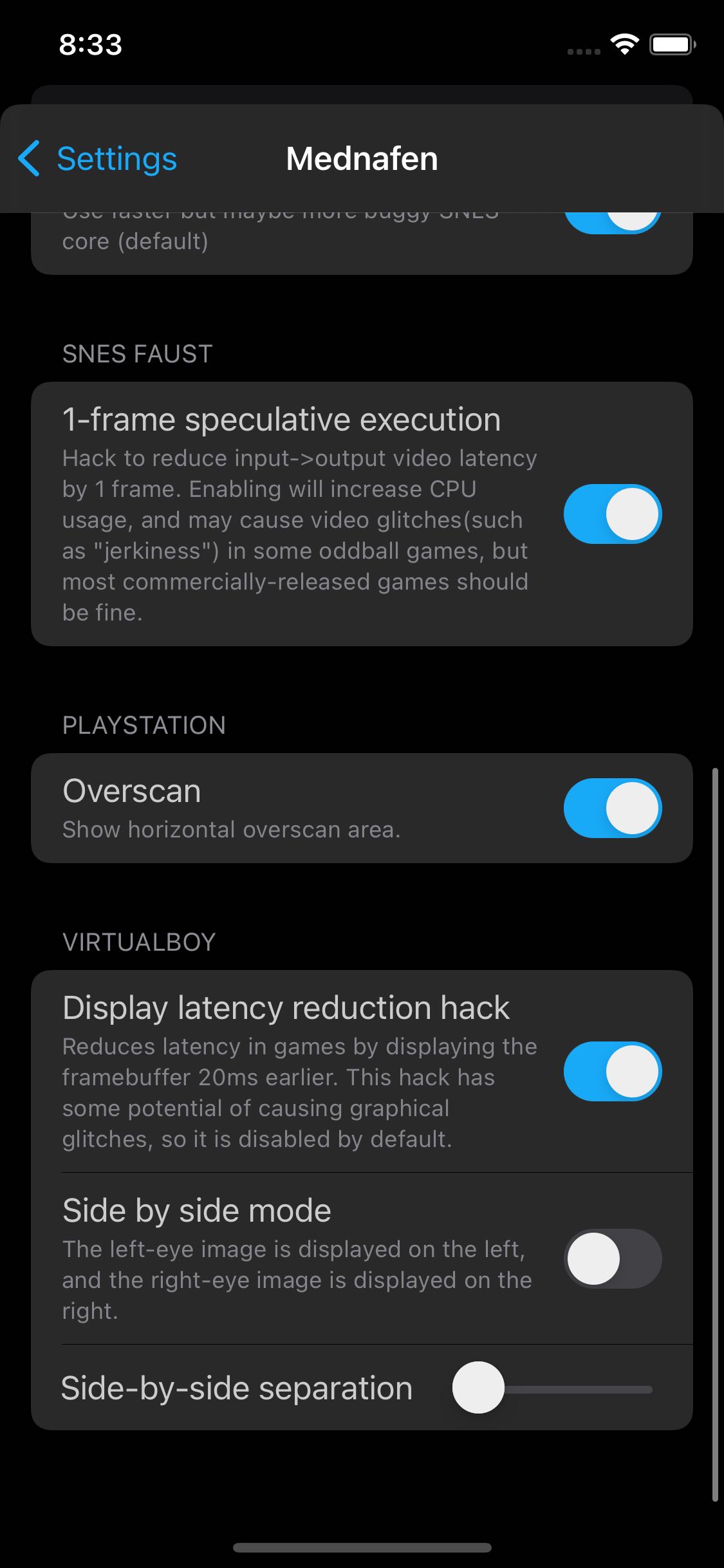The image depicts a webpage with a dark theme, featuring a black background and the time displayed as 8:33. In the top section, the web host information and a nearly full battery indicator are visible. As the viewer's eyes move down from left to right, the settings icon highlighted in blue is noticeable, followed by the word "MedNothin" prominently centered in the middle of the page.

The lower portion of the page appears somewhat blurred, and not all text is in English. Key phrases include "SNESFAST: one frame speculative execution," with a detailed explanation stating, "Hacked to reduce input-output video latency by one frame. Enabling this will increase CPU usage and may cause video glitches, such as jerkiness in some unusual games, but most commercially released games should be unaffected." To the right of this explanation, there is a blue and white indicator button, which appears to be activated.

Further down, there is a section labeled "PlayStation Overscan," with an option to "show horizontal overscan area," accompanied by another blue and white activated indicator button.

The following section addresses "Virtual Boy display latency reduction hack," which "reduces latency in games by displaying the frame buffer 20ms earlier. This hack may cause graphical glitches and is disabled by default." Another blue and white indicator button is to the right, which looks to be disabled in this context.

The final options relate to "Side by side mode," which explains that "the left eye image is displayed on the left and the right eye image is displayed on the right." The indicator button here is gray and white, signifying it is not activated. Lastly, there is a note about "Side by side comparison separation," featuring a white button that resembles a lever.

This webpage seems to be an interface for configuring various gaming emulation settings, each with detailed descriptions and toggles for activation.